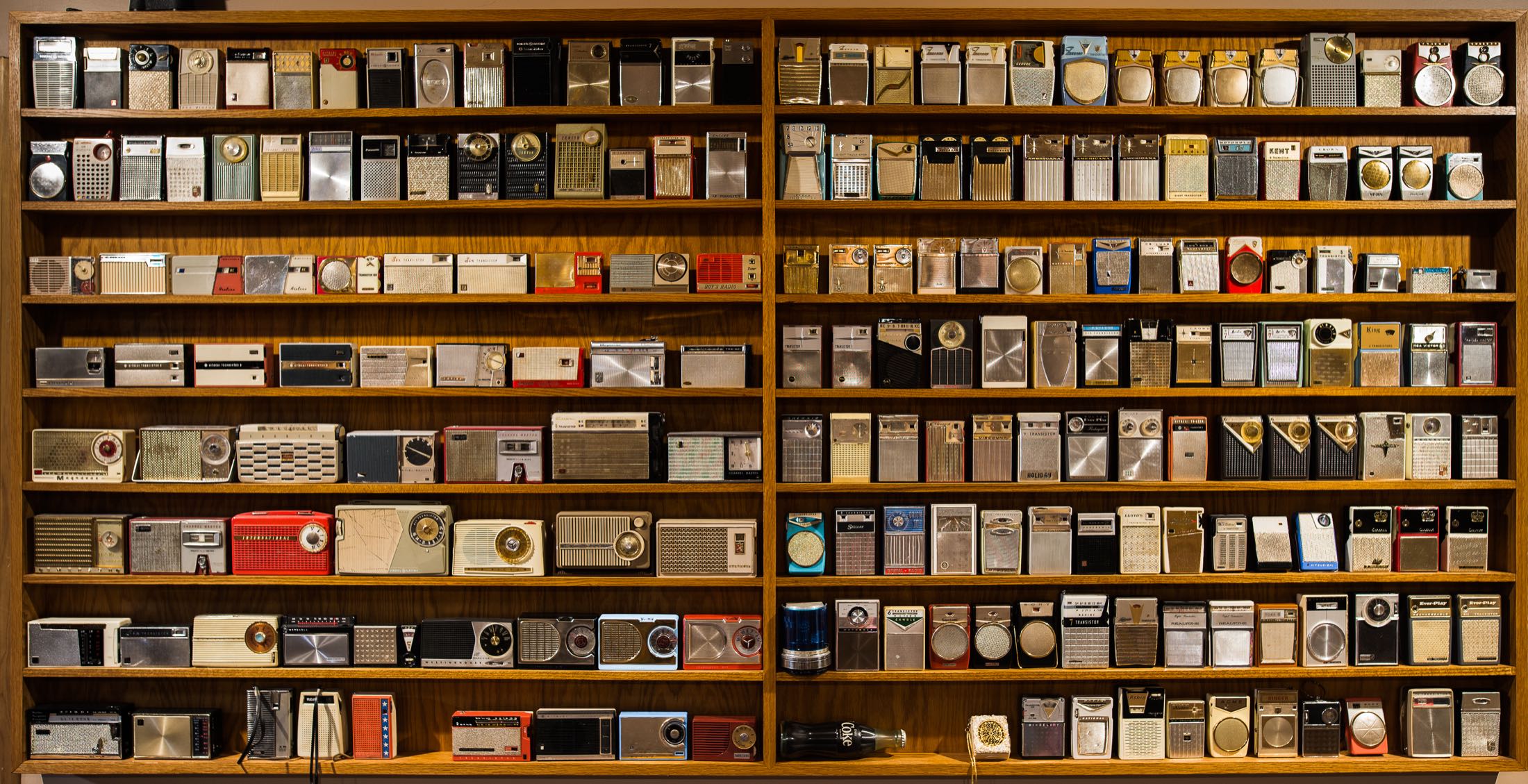The image features a large, brown, wooden bookcase with a metal divider at the center. The bookcase consists of two sections, each containing eight rows of shelves, making up a total of 16 rows. These shelves are filled with a variety of vintage radios, including old-school music speaker radios and potentially some clock radios. The radios come in various colors, such as reds, whites, and greens, and are meticulously organized by design. On the left section, higher shelves house smaller, rectangular, fridge-like radios, while the lower shelves display more vertically elongated models. On the right section, similar vintage radios fill the shelves. Notably, towards the middle bottom of the right section, a glass bottle of soda is positioned, lying flat. Additionally, a vintage calculator can be spotted in the top left corner. The overall arrangement showcases a stunning and meticulous collection of handheld radios spanning different eras, offering a nostalgic glimpse into the past.